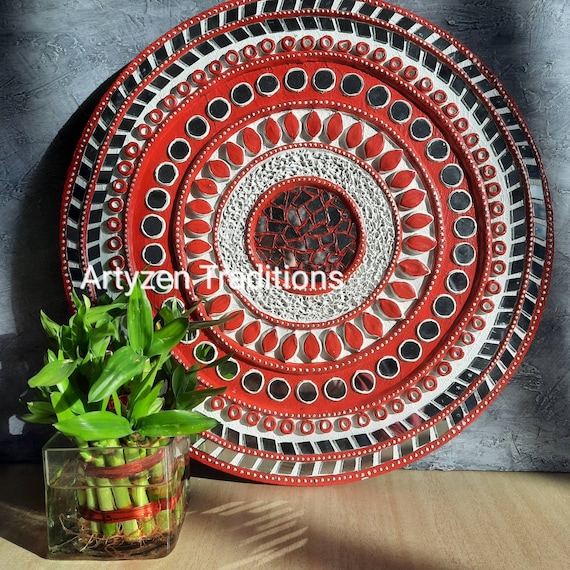The image showcases a detailed ornamental circular piece prominently displayed against a gray, natural textured stone wall. The decoration has an artisanal, possibly Native American or Aztec design, featuring concentric circles adorned with intricate patterns. The outer ring of the circle is embellished with small white dots and red rings, bordered by what appear to be square pieces of glass. Moving inward, there are red leaf shapes, black dots, and broken black pottery pieces forming a distinctive mosaic on a red background. The central circle is black, contrasting sharply with the surrounding designs.

The circular piece is placed on a light brown wooden table. To the left of this centerpiece, there is a square glass planter containing vibrant green bamboo stalks, some of which are wrapped in red bands. The image has a watermark at the top that reads "Art Zine Traditions" in white, suggesting the presence of artistic and cultural influences. The overall composition of the photo underscores a blend of traditional craftsmanship and natural elements.